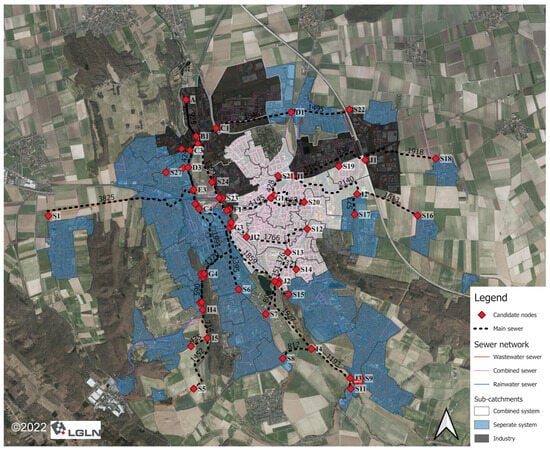The image is a highly detailed map of a city center surrounded by water and rural fields. In the center, white areas represent the city, marked with red diamond-shaped dots identified as candidate nodes in the legend, which is located in the bottom right corner. The map features various colored regions: blue, black, green, and grayish white, corresponding to different elements like sewer networks and subcatchments. The dotted lines indicate the main sewer network, with red lines for wastewater sewers, pink lines for combined sewers, and blue lines for rainwater sewers. Subcatchments are classified in the legend as white for combined systems, blue for separate systems, and gray for industrial areas. A direction arrow in the left of the image points upwards, and the bottom left is labeled "2022 LGLN." The map, with its abstract, almost mosaic-like appearance, combines an artistic style with detailed urban planning information.